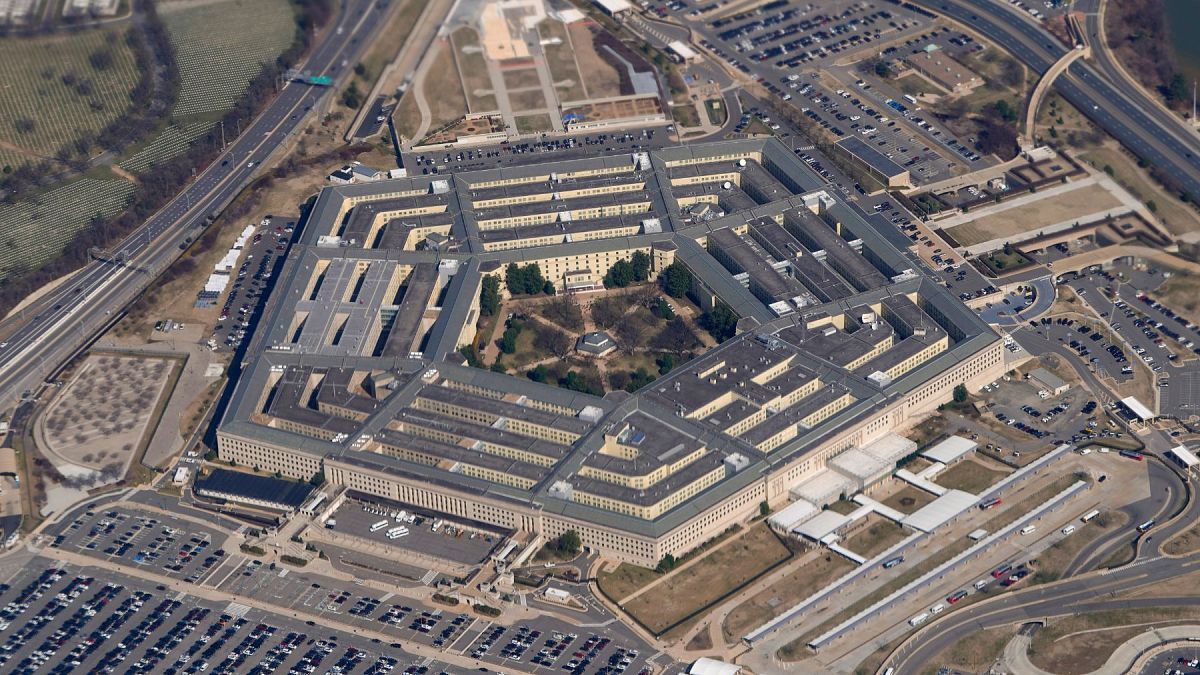The image is an aerial photograph of the Pentagon, taken from a high angle, possibly by a drone. The Pentagon, with its distinctive five-sided shape, is the main focus of the picture. Each side of the building is clearly visible, revealing the segmented structure with multiple strips indicating the separate sections within the complex. The walls of the Pentagon are white, while the roof appears gray.

In the center of the Pentagon, a courtyard garden is visible, featuring a gray fountain surrounded by tan walkways that extend out to each corner of the building. The courtyard is adorned with numerous bushes and trees, adding a touch of greenery to the otherwise beige and gray composition.

Surrounding the Pentagon on all sides are extensive parking lots, packed with countless automobiles. Major highways and roads snake around the Pentagon, particularly noticeable in the top left, top right, and bottom right corners of the image. In the distant background, smaller buildings are visible, which pale in comparison to the massive scale of the Pentagon.

The photograph appears to have been taken during the day, though it is not particularly bright. The orientation of the image has one of the Pentagon's points facing directly towards the viewer, offering a comprehensive view of the iconic structure and its immediate surroundings.